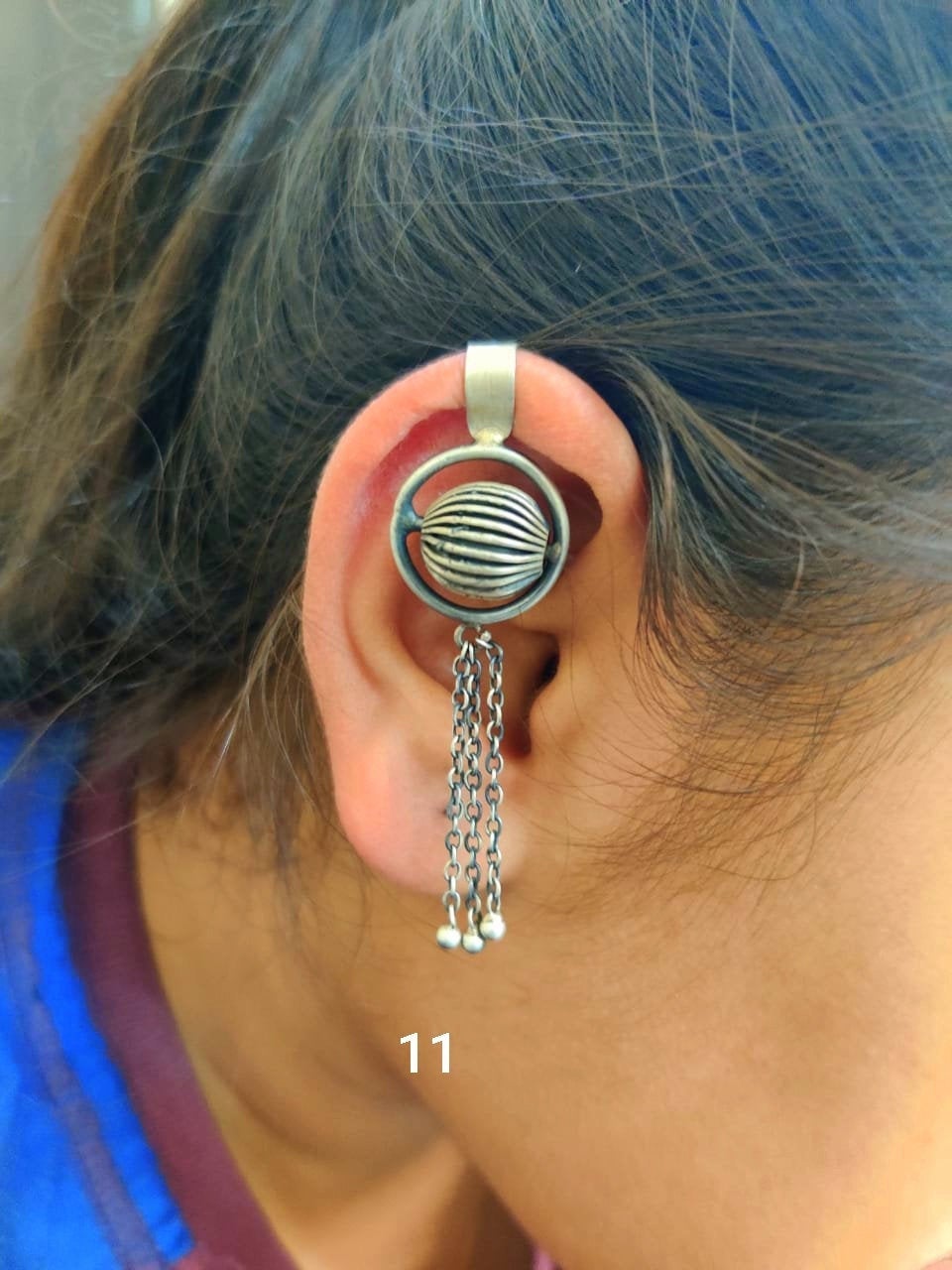The image is a close-up photograph mainly focused on a woman's ear, showcasing an abstract, metallic earring. The earring features a polished hoop with a central spinning ball that resembles a globe. Dangled from this hoop are three long chains, each ending with a small silver ball. The woman, with dark brownish-black hair tied in a ponytail, has tanned white skin. She is wearing a purple shirt under a blue coat. In white text below the ear, the number "11" is displayed, possibly indicating a product listing.